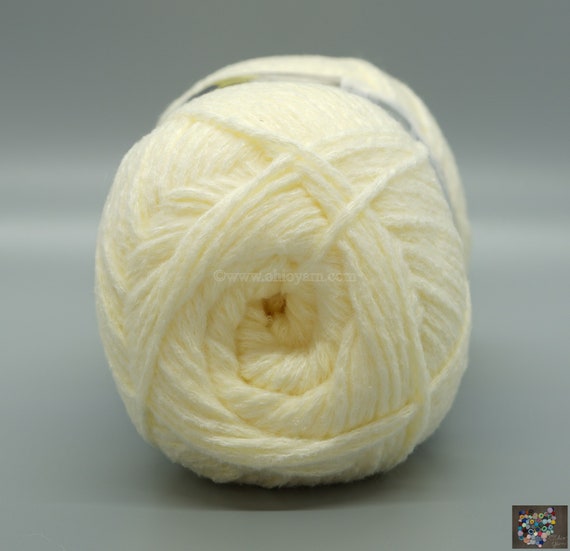The image features a small ball of light cream-colored yarn with a slight yellowish tint, suggesting a soft, silky, and fuzzy texture. The yarn appears thin, not chunky, and is spiraled neatly with multiple loops winding counterclockwise. A dark gray label is wrapped around the middle of the ball, providing contrast against the soft hue of the yarn. The yarn is positioned on a gray surface, and the entire background is a slightly blurry gray, offering a subtle, unobtrusive backdrop that keeps the focus on the delicate texture and intricate details of the yarn ball.